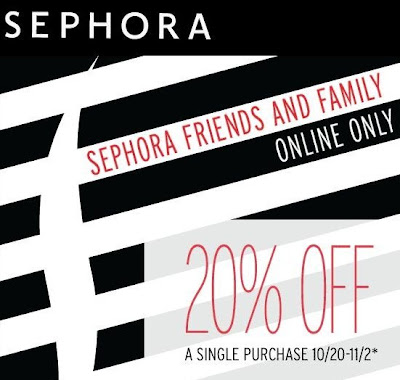The image is a Sephora advertisement promoting an online-only Friends and Family event. At the top, the word "Sephora" is prominently displayed in bold white letters on a black border. Below this, the background consists of angled black and white stripes, adding a modern and minimalist aesthetic that draws attention to the key information.

In the center, "Sephora Friends and Family" is written in striking red text, emphasizing the special event, while "online only" is placed in contrasting white text on one of the black stripes. Towards the bottom right corner, the coupon detail is clearly stated: "20% off a single purchase from 10/20 to 11/2," accompanied by an asterisk indicating potential exclusions or limitations.

The overall design is clean and visually appealing, with the classic Sephora logo—a stylized "S"—featured prominently. The minimalist black and white stripes background enhances the readability of the text and underscores the sophistication of the brand.